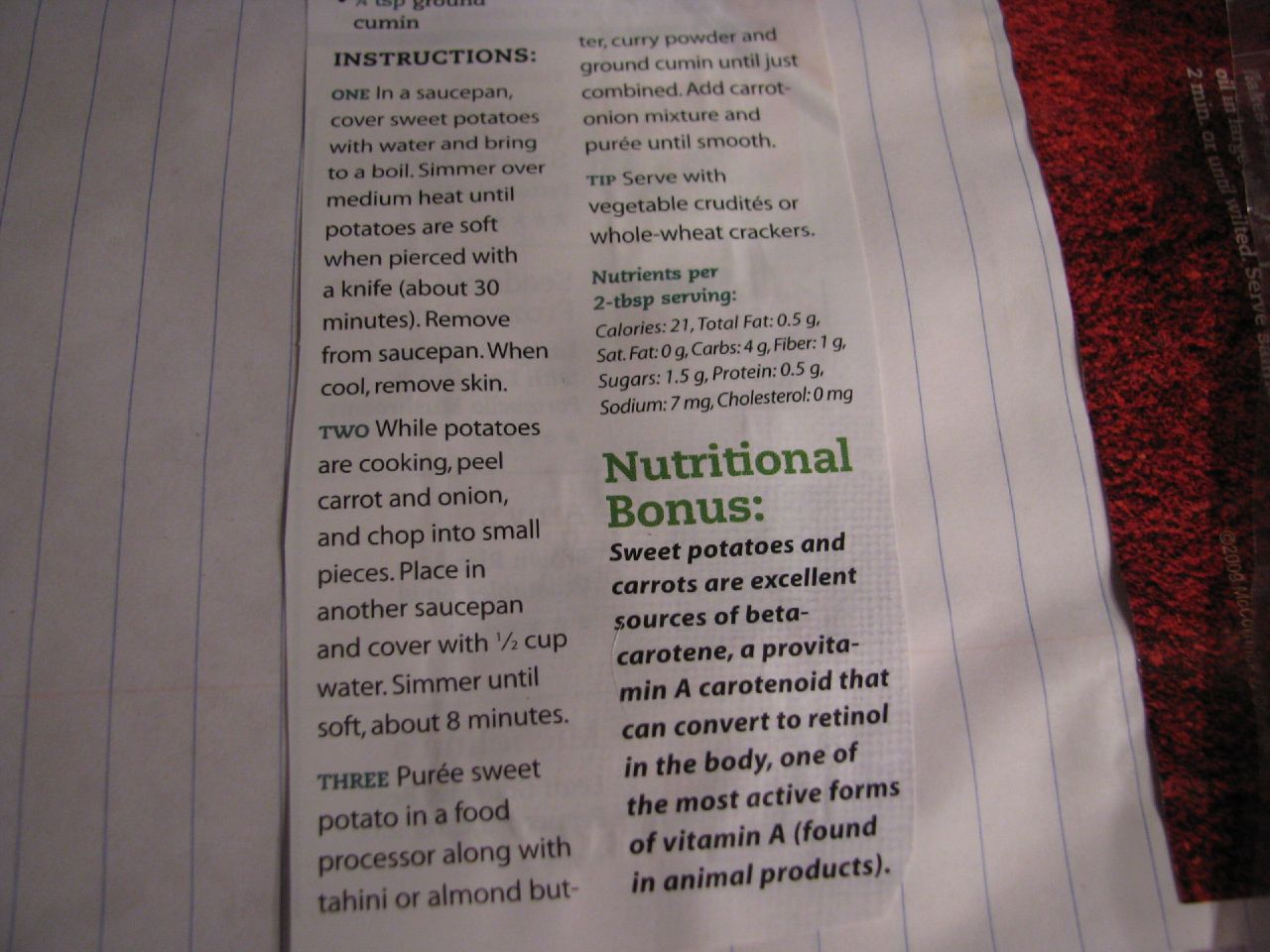In the right section of the image, a reddish-brown fuzzy surface, possibly a towel or carpet, is visible with hints of white beneath it. Atop this surface, a piece of lined paper lies sideways, with its light blue lines oriented vertically. Adjacent to the lined paper is a white sheet containing black printed text highlighted with green headers. The green header reads "Nutritional Bonus," followed by a description in black text: "Sweet potatoes and carrots are excellent sources of beta carotene, a provitamin A carotenoid that can convert to retinol in the body, one of the most active forms of vitamin A found in animal products."